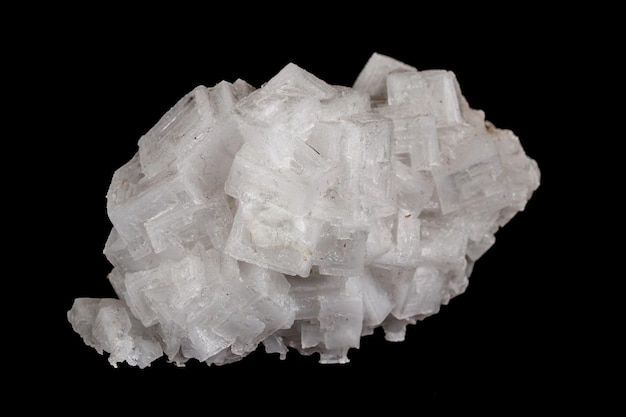This is a color photograph of a jagged, white mineral cluster, likely quartz or a salt crystal, set against a solid, black background with no text or light interference. The mineral takes up a significant portion of the horizontal, rectangular frame, appearing centered within the image. The cluster consists of numerous translucent, cube-like structures that form together to create a natural, unpolished shape. Its overall appearance is white, with some brown specks adding to the texture and shading. The crystals are more opaque at the center and become increasingly translucent towards the edges, giving it a layered and three-dimensional effect. The unique formation of the mineral gives it a fish-like silhouette, with the "head" on the right and the "fin" towards the back.